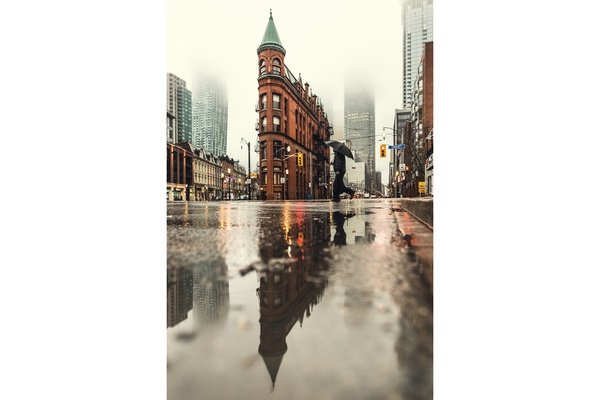The photograph captures a rainy street scene in Ontario, showcasing a blend of historic and modern architecture. Dominating the middle of the image is a tall, slender building with a conical, green oxidized copper rooftop, reminiscent of classic architecture yet surrounded by more modern skyscrapers. The camera angle, positioned low to the street, emphasizes the rain-soaked surface, which beautifully reflects the cone-topped tower, adding depth to the composition. A man carrying a dark umbrella walks across the street, highlighted by the reflections of red and yellow traffic lights on the wet pavement. The scene is set against a backdrop of a hazy, overcast sky, partially obscuring the tops of the surrounding buildings and contributing to the atmospheric feel of the photograph. Utility lines and the bustling urban environment frame the historic building, making it a striking focal point in this detailed and evocative cityscape.